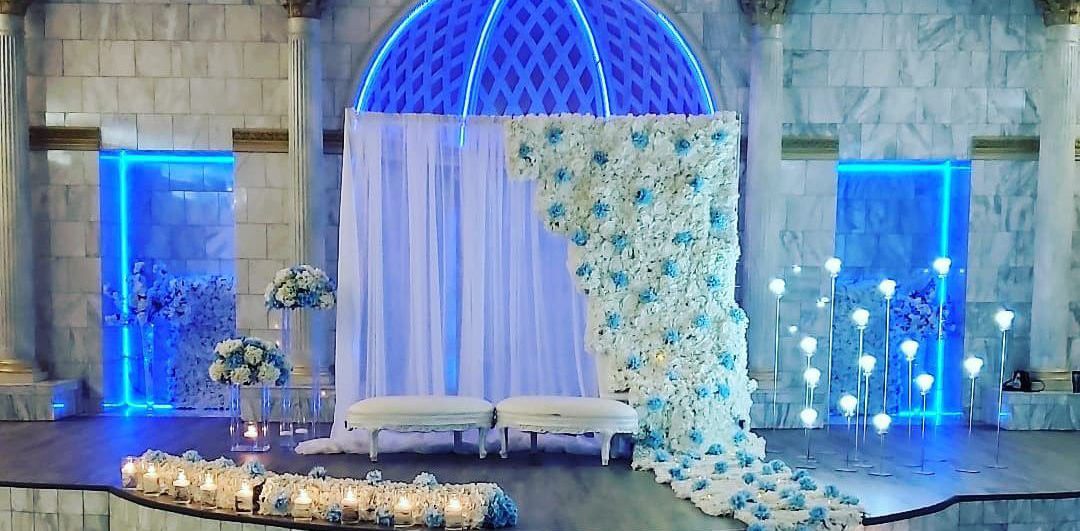The image captures a luxurious room with an ornate, dome-shaped lattice roof at the center, from which semi-circular curtains in varying shades of blue and white gracefully drape down to the floor. The floor, covered in a subtle gray tile, leads to a regal setting inside what appears to be a grand castle or a building fit for royalty. The walls are adorned with blue and white patterned wallpaper, and multiple marble pillars—some with gold bases and tops—stand tall around the room. 

On the right side, a heavier, flowery curtain is pulled back, revealing intricate fabric with white and blue dots hanging alongside. In front of these drapes, a white sofa and a series of different-sized floor lamps illuminate the space, casting a soft glow. There are also two elegant white benches flanking the curtained area, providing additional seating. 

In the background, two elevator-like doors outlined in neon blue light add to the modern yet opulent feel of the room. Between these doors stands a series of silver vases with white and blue flowers, further enhancing the sophisticated ambiance. To the left, an additional passageway suggests access to another room, while a distinct drop-off in the floor hints at the presence of a pool. This horizontal, rectangular photograph captures a blend of classical and contemporary design elements in a room exuding elegance and splendor.